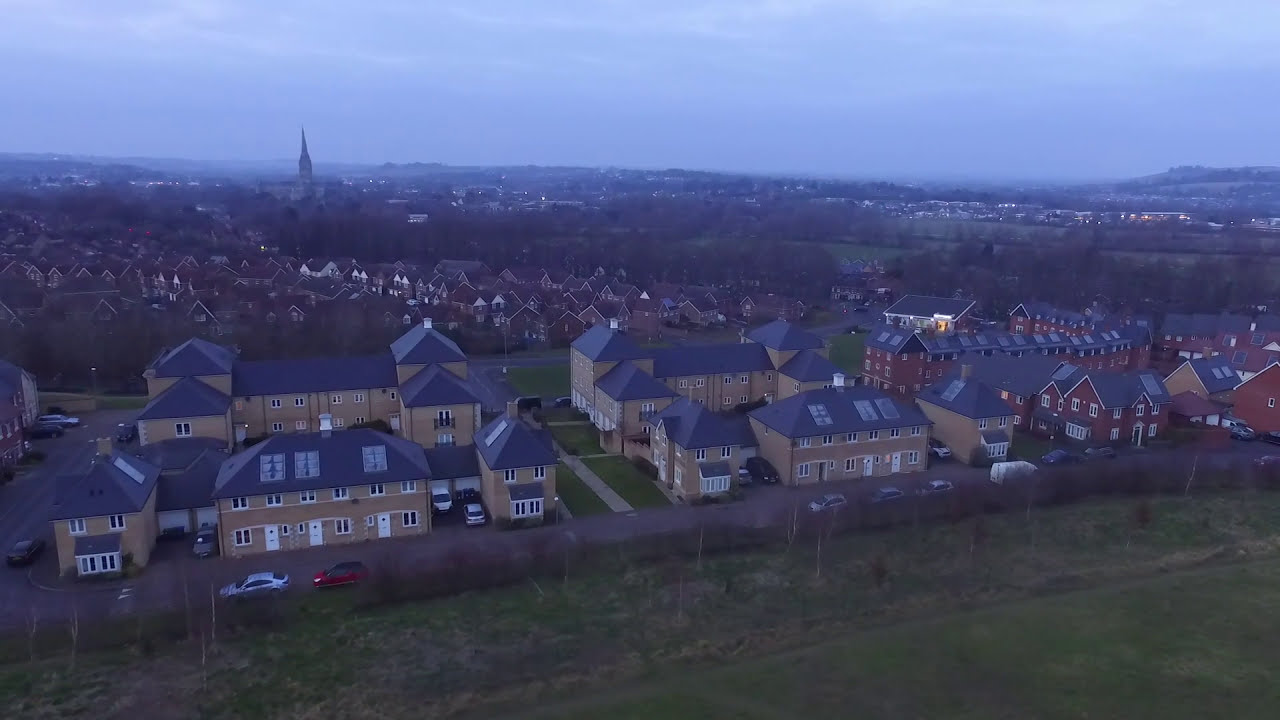This digital photograph captures an expansive townscape under a sky tinged with shades of pale blue, dark blue, and gray, suggesting the time is either dusk or early morning. The elevated view, likely taken from a drone, covers several blocks of multi-unit row houses in cohesive brown and red hues with slanted gray roofs featuring skylights. These homes share a uniform architectural style, nestled amid trees, cars, and fences lining the tranquil streets. The left portion of the scene is dominated by a prominent spire, possibly belonging to a church, rising above the rest of the buildings. The foreground includes a green, grassy field with low foliage and bushes, separated by a fence and followed by a road. The background reveals more houses and a hint of hills, enhancing the serene yet bustling atmosphere of the neighborhood.